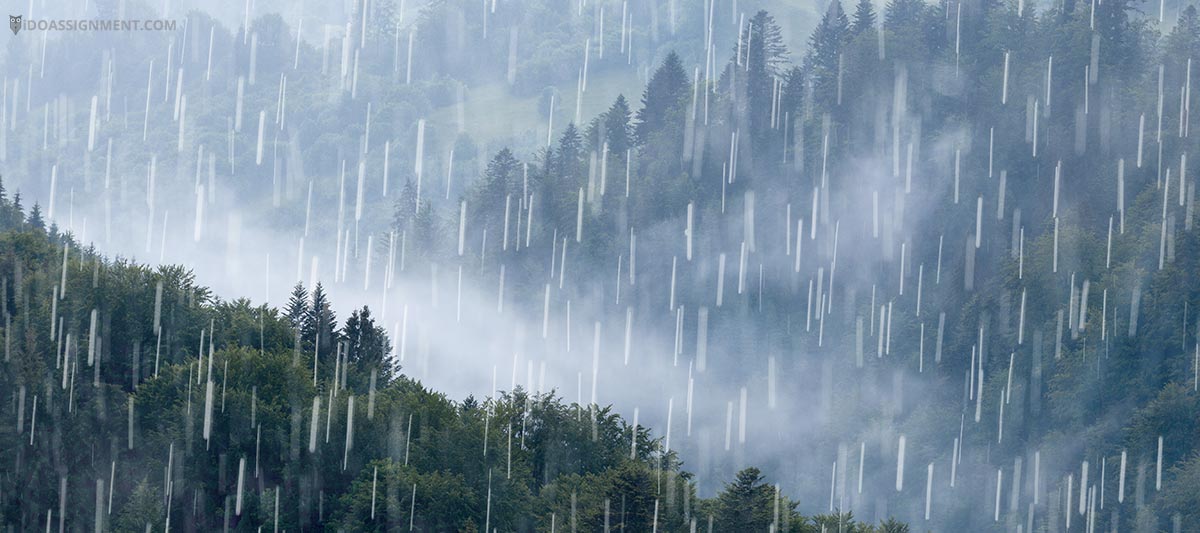The image depicts a dense forest or rainforest under an overcast sky, characterized by a heavy rainstorm. Two mountains converge into a fog-laden valley, suggesting a captivating, misty atmosphere. Raindrops cascade down in long, white streaks, capturing the motion of the downpour. The verdant landscape features a variety of thick, green trees, including dark and light green hues along with pine tree tips. In the background, there is a clearing that hints at a small field, lending depth to the scene. The entire image has a bluish tint due to the rain. In the top left corner, the text "IDOassignment.com" is accompanied by an owl icon, subtly marking the image.